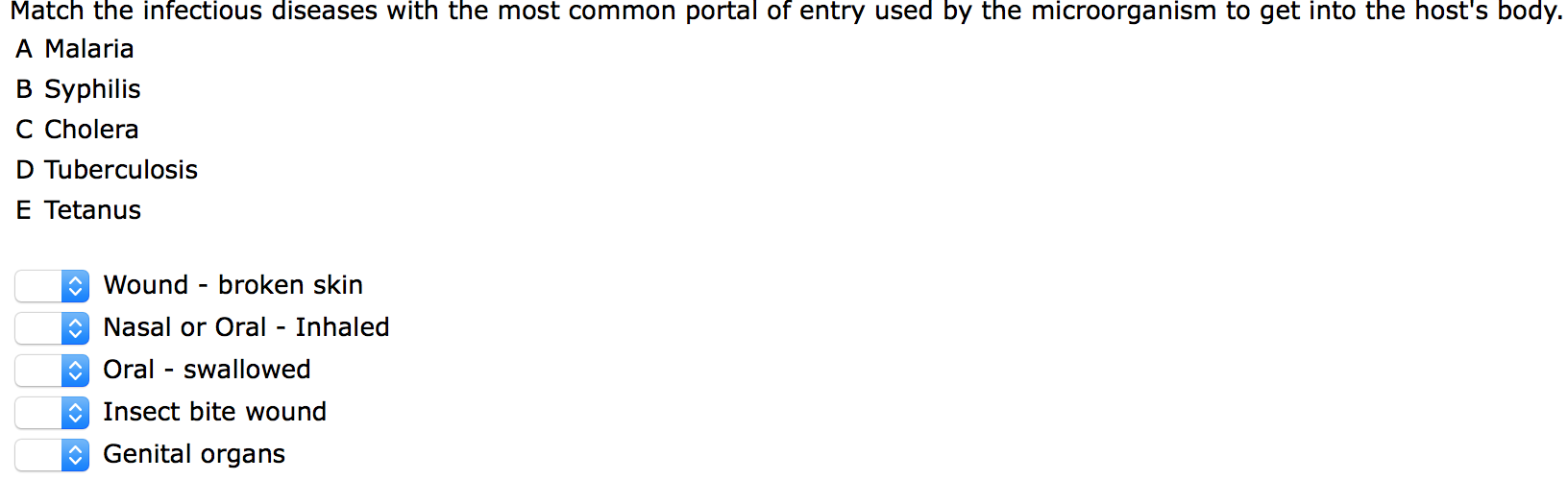The image features a clean, plain white background with black text and several interactive sections highlighted with a blue and white color scheme. At the top, a bold heading instructs the viewer to "Match the infectious diseases with the most common portal of entry used by the microorganism to get into the host body." Below this instruction, a list of infectious diseases is presented, including malaria, syphilis, cholera, tuberculosis, and tetanus.

Adjacent to each disease name, there are corresponding options for the most common entry points for these microorganisms. The options displayed are: wound/broken skin, nasal, oral (inhaled), oral (swallowed), insect bite wound, and genital organs. Users are prompted to match each disease with the appropriate portal of entry by placing the corresponding letter next to the correct option.

Clear and intuitive, the design ensures simplicity and ease of understanding, allowing users to focus on accurately matching diseases to their points of entry. The page is well-organized, devoid of extraneous details, making the task straightforward and minimizing potential confusion.